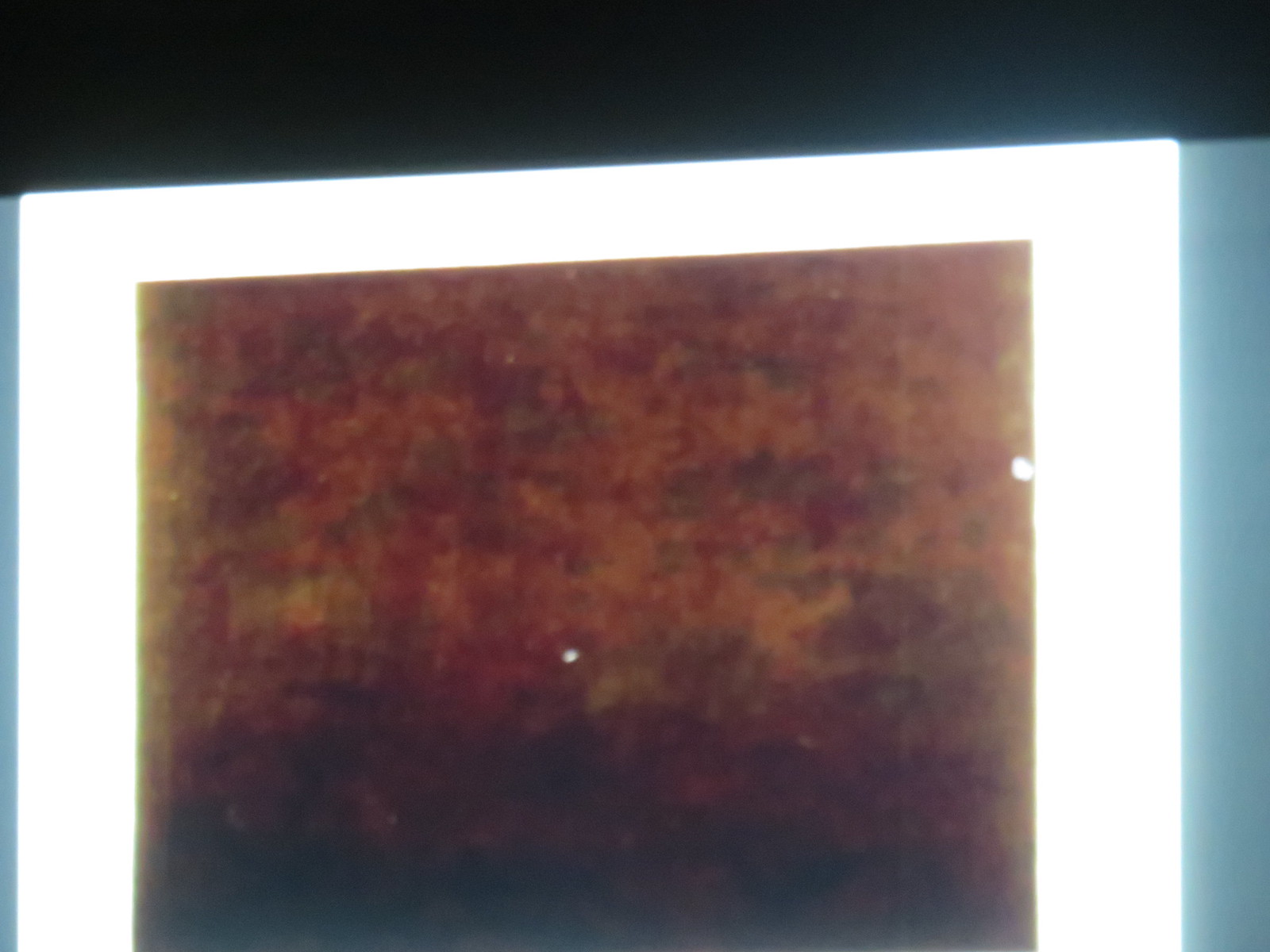The image features a central brown square with two white dots—one at the center and another slightly to the upper right. This brown square is framed by a large white square, which in turn is bordered by an incomplete blue square visible only on its left and right sides. The entire composition rests against a black background, giving the appearance of an x-ray or backlit document. The brown square has a contrast of black and fades from darker shades at the bottom to lighter shades towards the top. The setting seems to be in a dark room with the background light enhancing the vivid colors and details of the brown square. This illuminated effect possibly resembles photographic development processes, although the bright light diverges from the typical red lighting used to develop photos. Overall, the arrangement and lighting give a detailed and striking visual contrast.